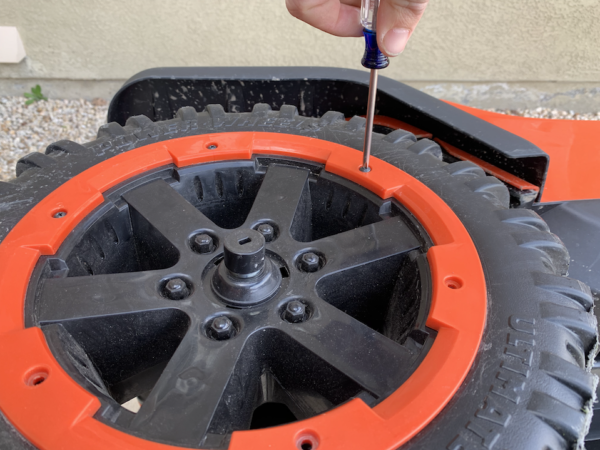In this image, a Caucasian individual is using a small metal screwdriver to insert a silver screw into an orange circular base encircling a black wheel that is positioned sideways. The black wheel features visible black bolts around its base and a plastic rim inside. The back wall is an oatmeal color, and the ground to the left and slightly to the right is covered with white and grayish pebbles. An orange lip, shaped almost like a flat V, extends over the black wheel base. There are black font letters on the wheel, spelling out "ULTMAT."